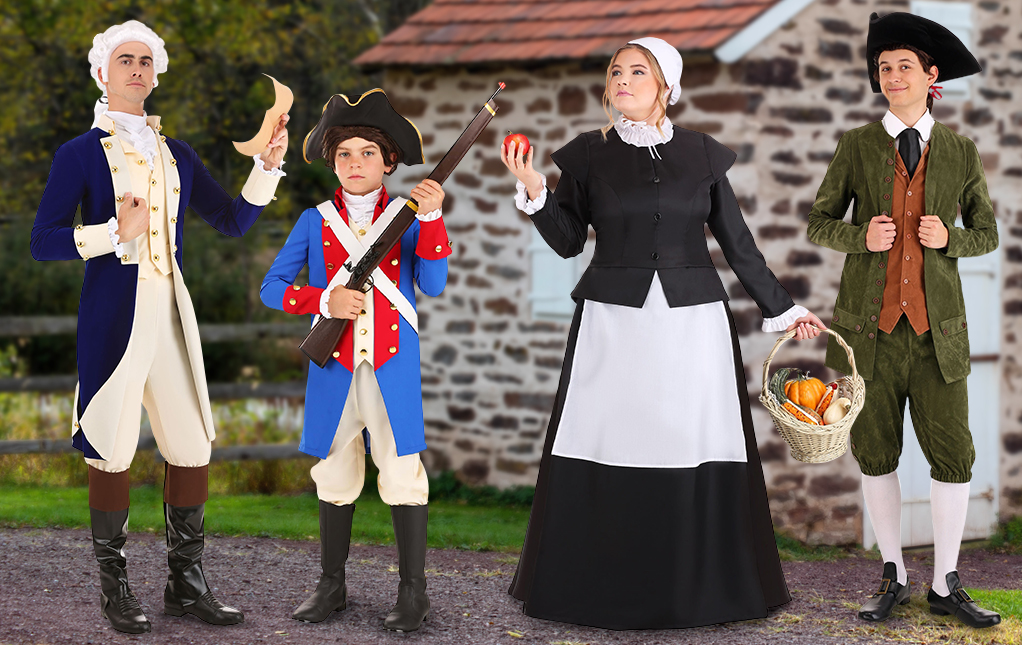In the photograph, four individuals dressed in meticulously accurate 18th-century colonial attire pose in front of an old stone cabin. The central figure is an adult man clad as an American founding father, complete with a white wig, a blue jacket, a cream-colored vest and matching pants, and black riding boots. He holds up a piece of parchment, likely meant to represent the Declaration of Independence. To his right stands a young boy, distinguished by his three-cornered hat, red, white, and blue jacket, tan pants, and black boots. He carries a musket, adding to the historical authenticity. Further to the right, a woman appears, wearing a black coat over a long black skirt, a lace choker-style necklace, a white apron, and a white bonnet. She holds up an apple and carries a basket full of period-appropriate vegetables. Finally, on the far right, is a young man in a green suit with a brown vest, green pants, white socks, and buckled shoes, all topped with a three-pointed hat. Together, they create a vivid tableau of colonial American life.